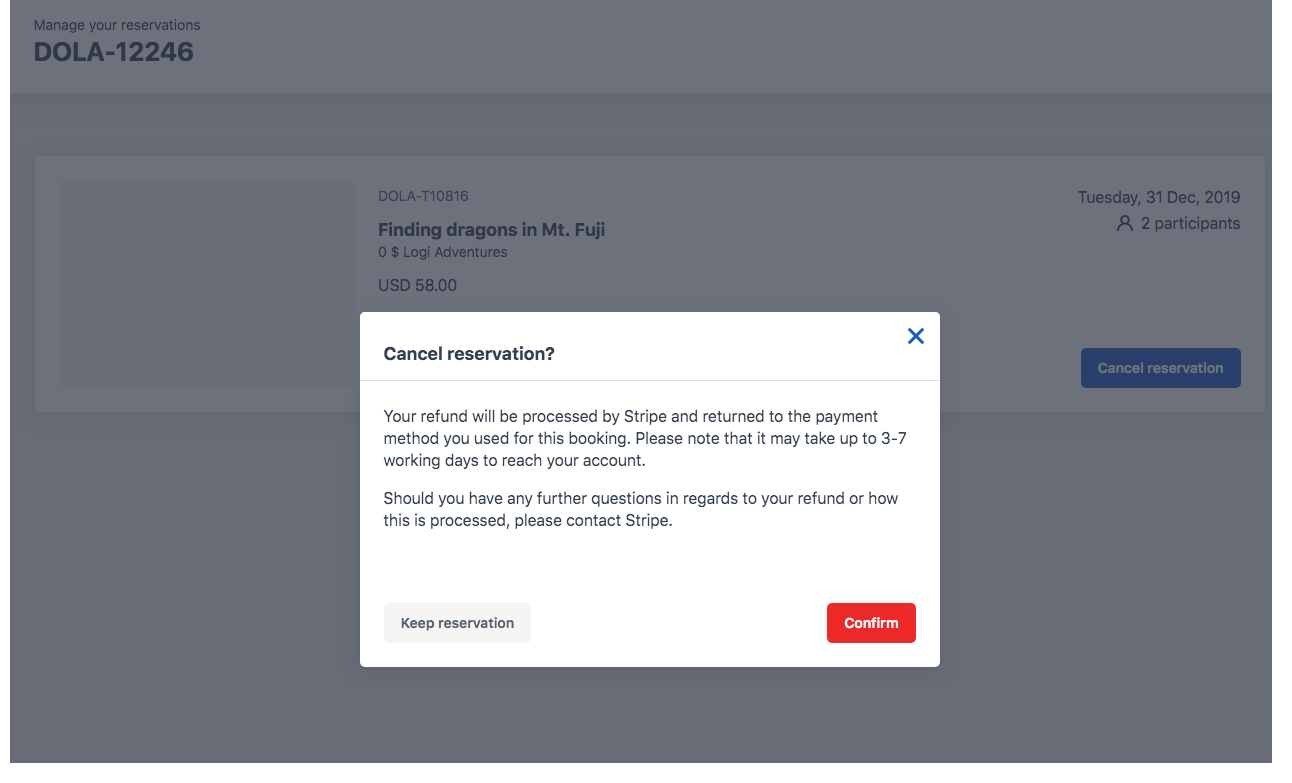In the expansive gray background of the interface, prominent text in the upper left corner reads "Manage Your Reservations." Below this, two alphanumeric codes are displayed: "DOLA-12246" and "DOLA-710815." 

Directly beneath these codes is the title "Finding Dragons in Mount Fuji," followed by the word "Adventures" and a price of "USD $58." 

Dominating the center of the screen is a large white square containing the text "Cancel Reservation?" Approximately five inches to the right of this square, there is an "X" icon to close the window.

Within the white square, additional information reads: "Your refund will be processed by Stripe and returned to the payment method you used for this booking. Please note that it may take up to three to seven working days to reach your account. Should you have any further questions regarding your refund or the process, please contact Stripe."

To the left of the "Cancel Reservation?" text, within a light gray rectangle, is the option "Keep Reservation." About five inches to the right of this option is a small red rectangle containing the word "Confirm."